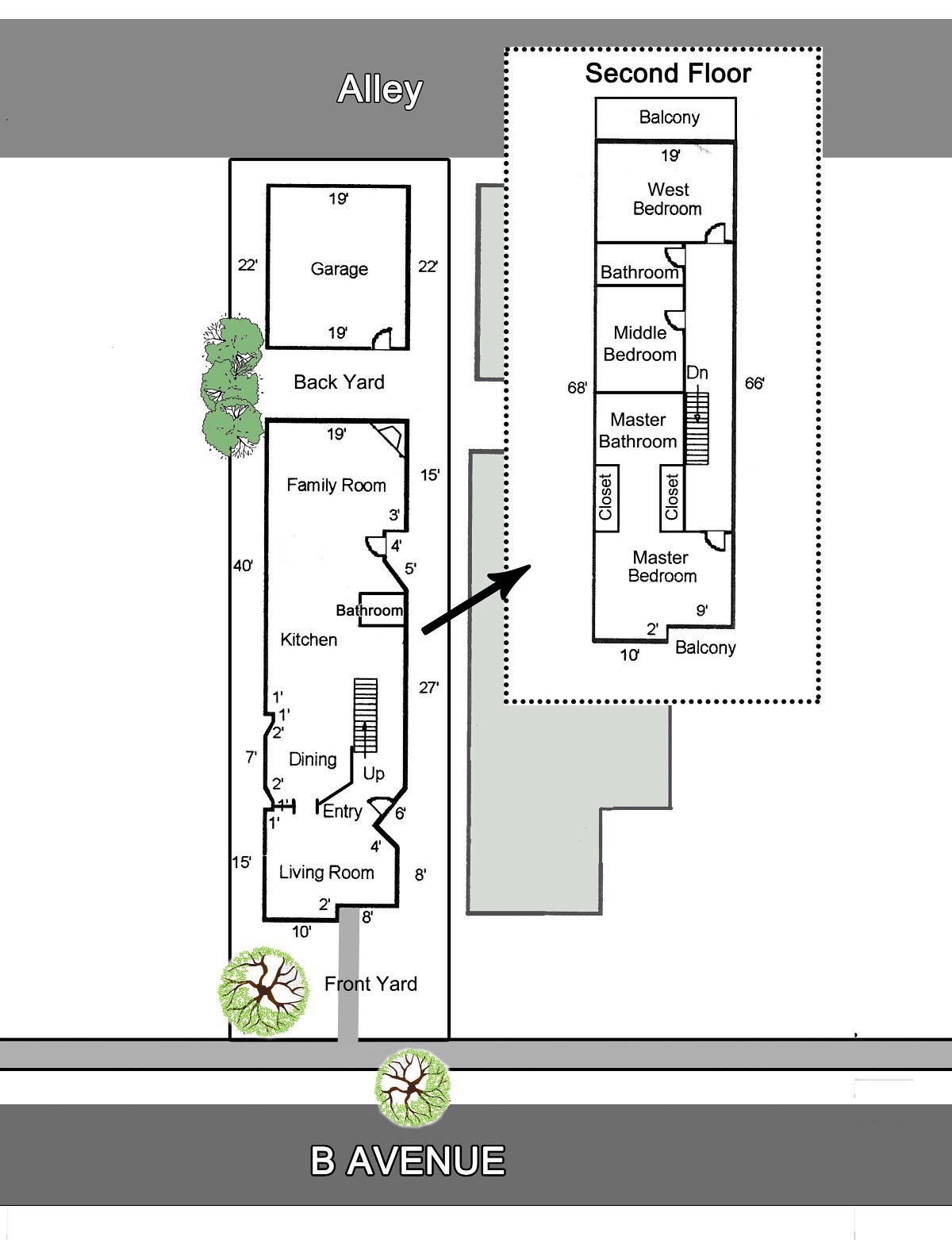**Detailed Diagram of a Two-Story House**

This meticulously detailed diagram shows a two-story home, bordered by ALLEY at the top and B AVENUE at the bottom. Each label is presented in bold, white font with a thin black outline; ALLEY is set on a black rectangular background, while B AVENUE is displayed on a darker gray rectangular background.

**Ground Floor:**
- **Garage:** Positioned on the bottom story, this 19 feet by 22 feet garage sits adjacent to the backyard.
- **Family Room:** Measuring 19 feet, the family room is directly connected to the garage.
- **Small Bathroom:** Located off to the right side, below the family room.
- **Kitchen & Dining Room:** Positioned centrally, the kitchen flows seamlessly into the dining room.
- **Entry & Living Room:** The entrance leads into a spacious living room.
- **Stairs to Second Story:** Situated to the right of the dining room, these stairs provide access to the upper floor.

**Second Floor:**
- **Balcony:** Features prominently at both the top and bottom of the second-floor diagram.
- **West Bedroom:** Located at the top, this bedroom is 19 feet wide.
- **Small Bathroom:** Situated to the left of the west bedroom.
- **Middle Bedroom:** Located adjacent to the small bathroom.
- **Master Bathroom:** Positioned on the left side.
- **Master Bedroom:** Found at the bottom of the diagram.
- **Hallway:** Housing the stairs that lead down to the first floor, the hallway runs along the right side of the diagram.

This diagram succinctly illustrates the comprehensive layout of the two-story home, offering clear dimensions and spatial relationships between the various rooms and features.